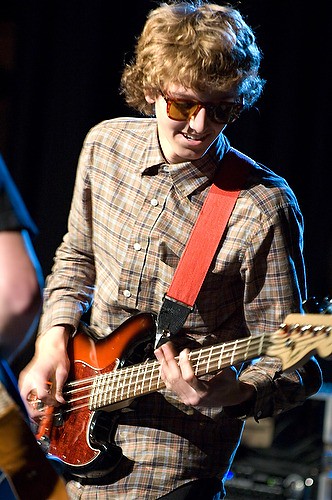The photograph depicts a young white man with shaggy, light brown or dirty blonde hair, wearing light brown sunglasses. He is dressed in a button-up collared shirt with a pattern that combines tan, blue or gray, and white stripes. He is energetically playing a reddish-brown electric guitar with a light brown to black gradient finish, which has a distinctive red strap over his left shoulder with a black part that hooks onto the guitar. His fingers are blurred in motion, suggesting a lively performance. To the left of the image, an arm of another individual, presumably another musician, is visible, wearing a black t-shirt. In the bottom right corner, some music or recording equipment, possibly a speaker or amplifier, can be seen. The background is completely black, which contrasts sharply with the well-lit subject and highlights the energetic scene being captured.